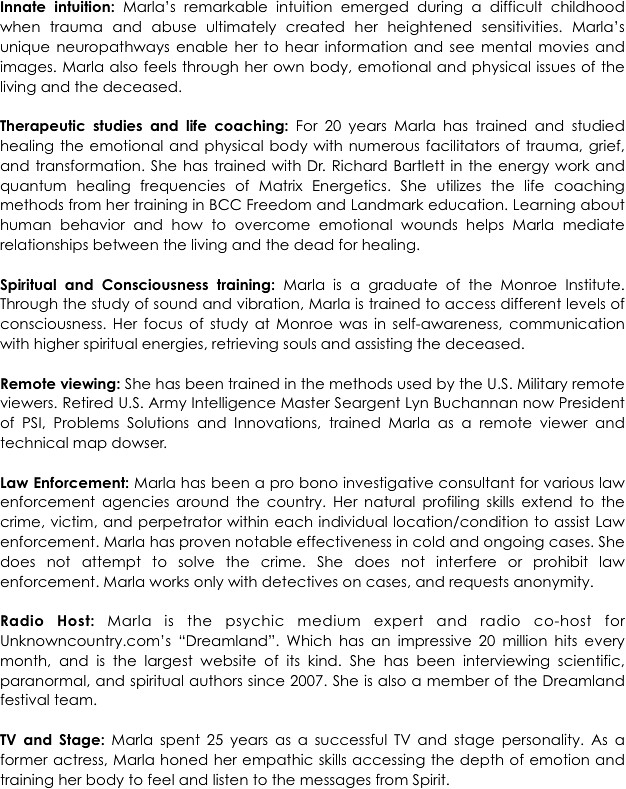The image showcases a detailed profile of a woman named Marla against a white background, filled with black text where key headings are in bold. At the top, the text "Innate Intuition" stands out, highlighting Marla's remarkable intuition that emerged from childhood trauma and abuse, enabling her unique neuropathways to perceive information through hearing and visualizing mental images. There are seven paragraphs, each marked by bold headlines that delve deeper into Marla's diverse expertise and experiences. 

1. **Innate Intuition:** Describes how Marla's heightened sensibilities allow her to feel emotional and physical issues.
2. **Therapeutic Studies and Life Coaching:** Details Marla's 20 years of training and studying the healing of the emotional and physical body under various facilitators specializing in trauma, grief, and transformation.
3. **Spiritual and Consciousness Training:** Notes Marla's graduation from the Monroe Institute, underscoring her proficiency in spiritual fields.
4. **Remote Viewing:** Mentions her training by the U.S. military, showcasing her skills in perceiving distant or unseen targets.
5. **Law Enforcement:** Indicates her involvement in law enforcement, though specifics aren’t provided.
6. **Radio Host:** Suggests her experience as a radio host, implying strong communication skills.
7. **TV and Stage:** Highlights Marla's 25 years as a successful TV and stage personality, where she honed her empathic abilities and trained her body to grasp and convey deep emotions, enhancing her understanding of societal messages.

Overall, this extensively describes Marla's multifaceted career and her profound abilities stemming from her intuitive and empathetic skills.